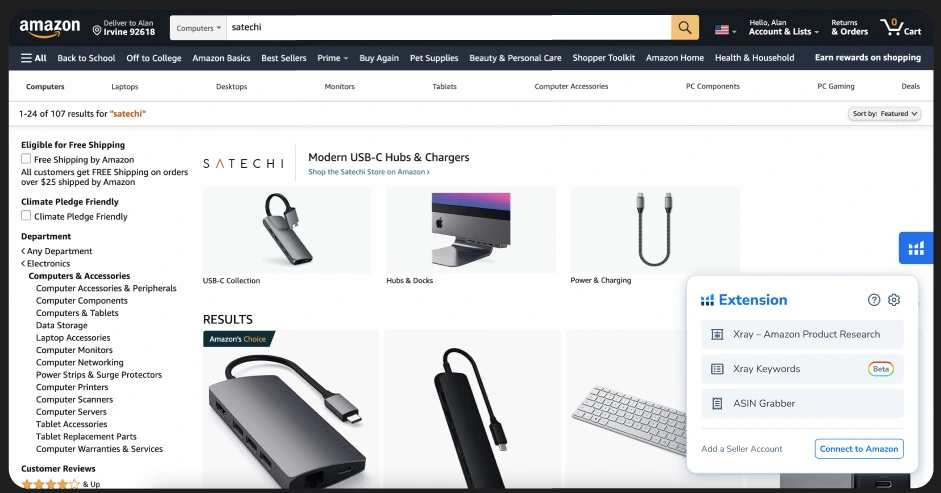This is a detailed and cleaned-up caption for the provided image:

"A cropped screenshot of the Amazon web page in desktop view is displayed. At the top left corner, the iconic Amazon logo is visible. To its right, there is the text 'Deliver to' followed by a city and zip code displayed in bright white text. Adjacent to this is the centrally positioned search bar. The search bar features a drop-down box on the left, set to 'Computers,' and contains the search term 'set techie.' The background of the web page is white. Towards the top left of the body, it shows '1 out of 24 of 107 results for so touchy.' On the bottom right, there is a small white pop-up box labeled 'Extension.' The top left corner of this box offers three options in gray boxes: 'X-Ray Amazon Product Research,' 'X-Ray Keywords,' and 'ASIN Grabber.' At the bottom right of the pop-up box, there is a button labeled 'Connect to Amazon.'"